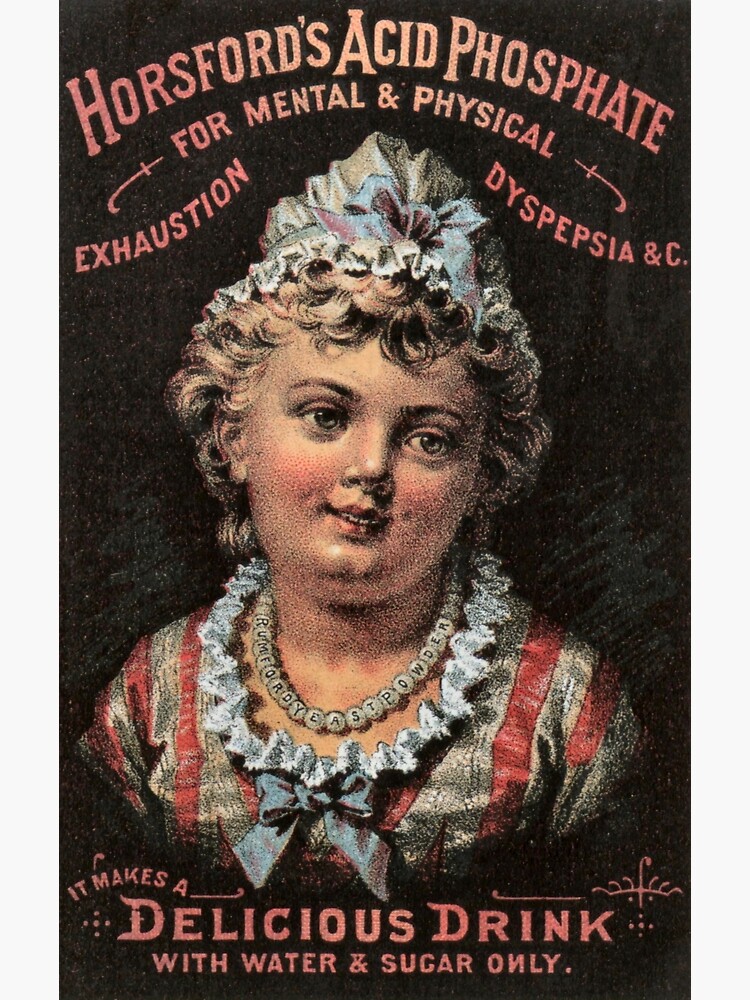This vintage poster from the late 19th or early 20th century is an advertisement for "Horsford's Acid Phosphate for Mental and Physical Exhaustion, Dyspepsia, and C." The poster features a painted image of a young girl wearing a nightcap and a playful grin on her face. She is dressed in a red and white striped shirt adorned with a frilly white collar and a blue bow. Around her neck, she wears a necklace with letters on it. The background is black, and the text at the top is stylized in an orangey-red hue. Below her image, the caption reads, "It makes a delicious drink with water and sugar only."